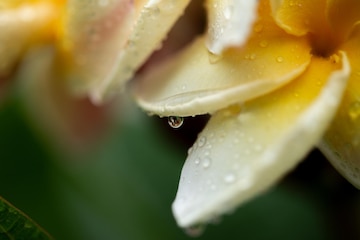The image is a highly detailed, close-up photograph of yellow and white flower petals, revealing intricate details typically not visible to the naked eye. The petals are adorned with shimmering droplets, suggesting a recent rainfall or watering. One prominently captures a pool of water near its flattened edge, poised with a tiny droplet on its verge, ready to descend. Above this, another petal contributes its own drip, creating a cascading effect that adds a dynamic quality to the scene. The photograph, likely non-digital, focuses so intimately on the petals that the larger form of the flower escapes recognition. Only a blurry hint of green in the background suggests foliage, set against an otherwise deep and darkened backdrop, enhancing the vividness and texture of the water-laden petals.